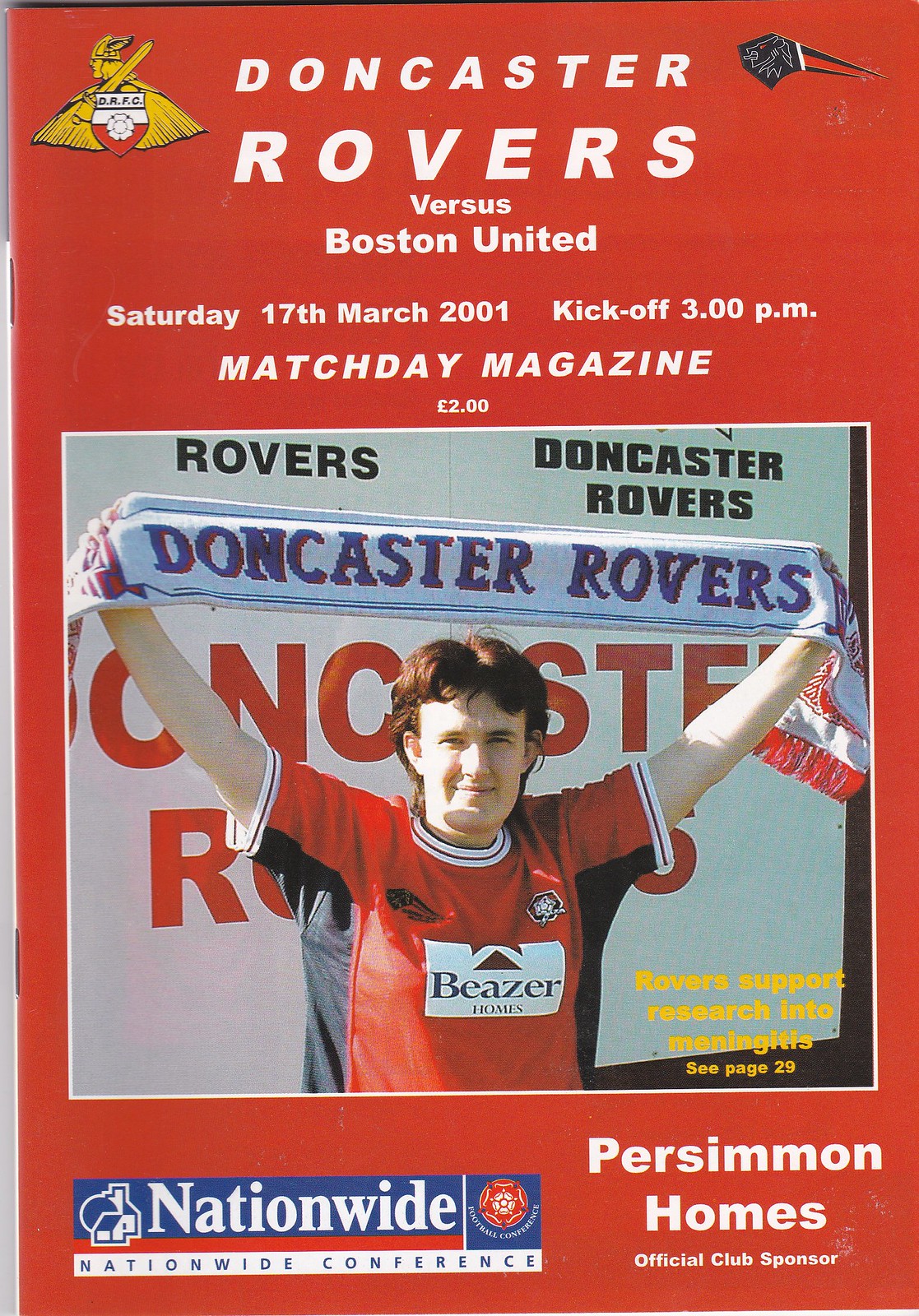The image features a vibrant red soccer program adorned with various details and iconography. At the top, in bold white font, it reads "Doncaster Rovers vs. Boston United, Saturday, 17th March 2001, kickoff 3:00 p.m. Match Day magazine, £2.00". Flanking the text are two icons: a golden soldier on the left and a lion's head on the right. Dominating the lower half of the cover is a full-color rectangular photo of a Caucasian male soccer player with wavy brown hair, dressed in a red and black jersey with "Beezer Homes" emblazoned in white on the chest. The player is holding a white scarf with blue text that reads "Doncaster Rovers", standing behind a banner that repeats "Doncaster Rovers" in black and red text. In the lower right corner of the photo, in small yellow print, it states "Rovers support research into meningitis. See page 29." At the bottom of the program is an advertisement for the "Nationwide Conference" and the phrase "Persimmon Homes official club sponsor" in the right corner.